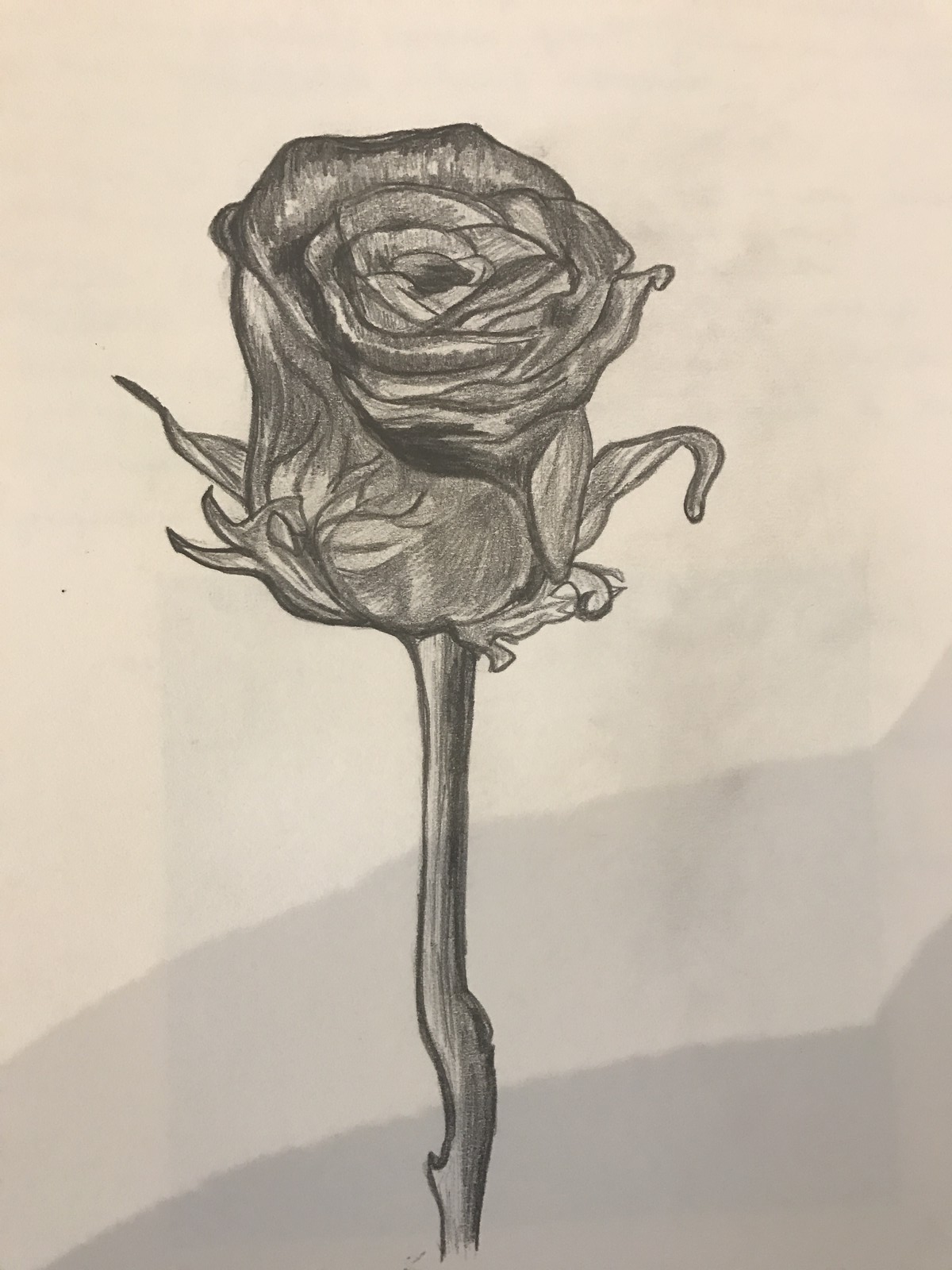This image is a photograph of a detailed graphite pencil drawing on a white sheet of paper, portraying a beautifully shaded rose. The top three-fourths of the page remains white, transitioning to light gray in the middle, and finally dark gray in the bottom portion, especially in the lower corners. The rose drawing extends from the bottom middle upwards, featuring a long, slender stem that appears slightly jagged, hinting at thorns. The stem supports the flower bud, which is slightly open, showcasing a tightly clustered arrangement of layered petals with an opening in the center. At the base of the flower, several small, almost triangular leaves are drawn, adding to the intricate detail. The shading and blend of pencil work add a three-dimensional quality, giving depth and dimension to the rose and its petals. The overall image captures the delicate and realistic essence of a blooming rose with meticulous attention to shading and detail.